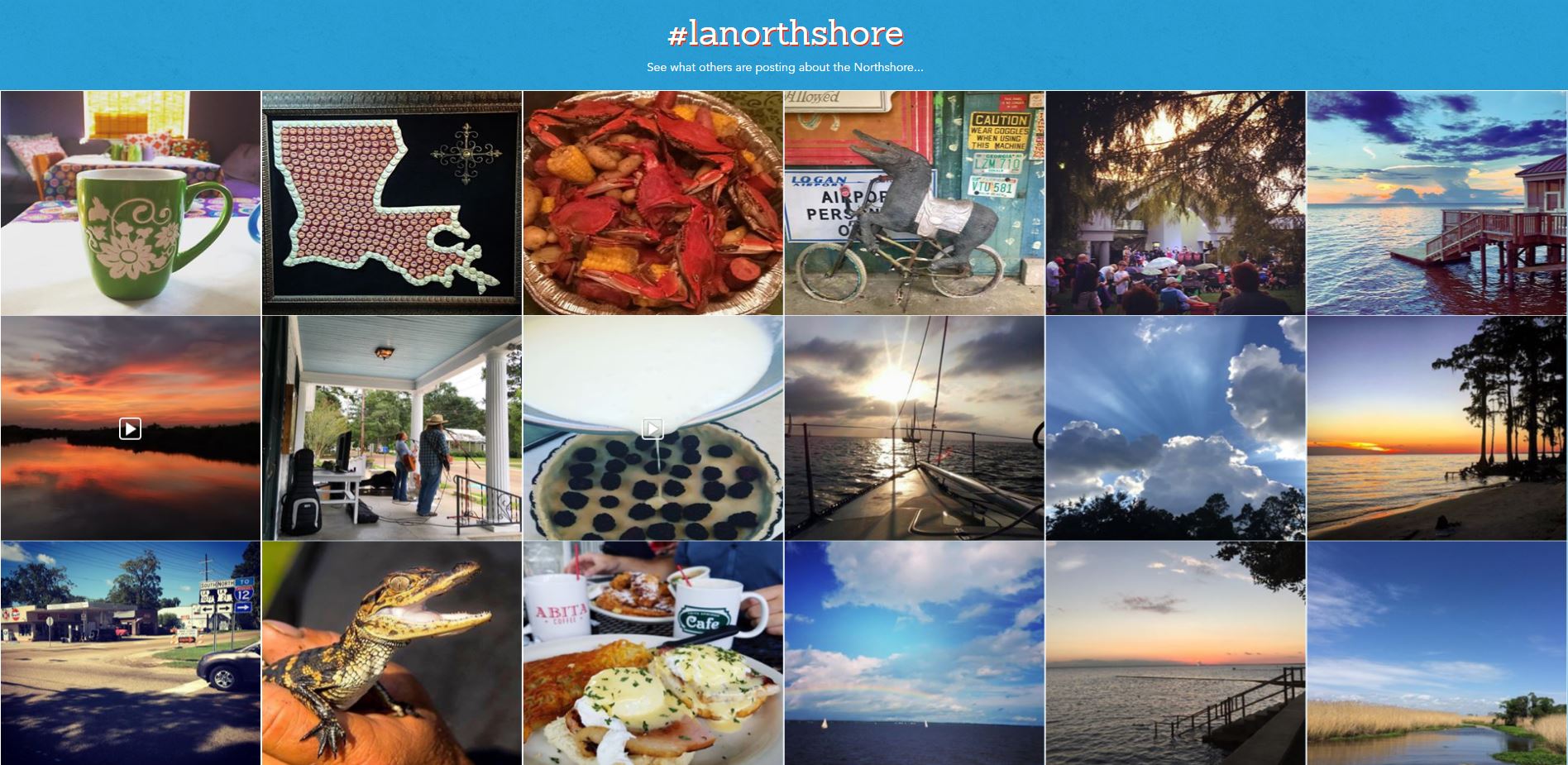The image is a collage of 18 photographs arranged in three rows of six, each showcasing various scenes and objects, most likely related to a specific destination, possibly Louisiana. The collage is titled "LA North Shore" or "Number or Tag L.A. Law of Soar," indicated by the text at the top. Prominently featured is a green coffee cup with a flower pattern on a white table in the top left corner, and nearby are images of a red map in the shape of a bush, a plate of crabs, and a bicycle with a toy animal. Additionally, there are scenes of a group of people in front of a white building, a house with steps leading to water, and a street with a black car. Further details capture a hand holding a lizard, a breakfast plate with ham and potatoes, and idyllic landscapes including a blue sky with clouds, an ocean, a flight of stairs, and a river flanked by blue skies and banks on each side. The collage encapsulates vibrant colors such as blue, yellow, red, black, green, and orange, emphasizing a scenic and diverse region.